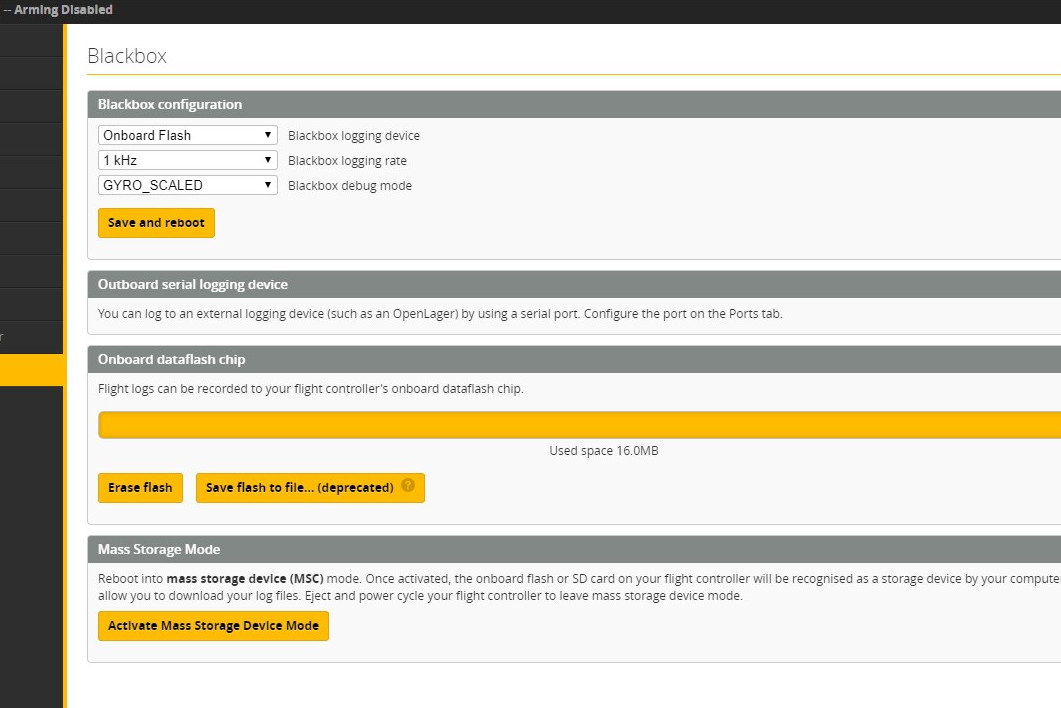The image is a horizontally rectangular screenshot featuring a comprehensive interface for a flight controller's black box configuration. The outer border of the image is black, with "arming disabled" text prominently displayed in the top left corner. The majority of the screenshot comprises a white background adorned with various sections enclosed in light gray boxes, each with a dark gray border and heading.

The initial heading at the top reads "Black Box" followed by "Black Box Configuration," which houses drop-down menus for configuring the logging device, logging rate, and debug mode. Below these options, a teal-colored "Save and Reboot" button is available for saving changes.

The next segment is titled "Outboard Serial Logging Device" and contains instructions for logging data to an external device via a serial port, directing users to configure this port on the "Ports" tab.

Following this is the "Onboard Data Flash Chip" section, which allows users to record flight logs to the flight controller's onboard data flash chip. An entirely yellow bar beneath this section indicates "Used Space: 16MB." Options to "Erase Flash" and "Save Flash to File" are provided below the usage bar for managing the data flash chip.

The final section is "Mass Storage Mode," featuring a single button labeled "Activate Mass Storage Device Mode" for switching the device to mass storage mode.